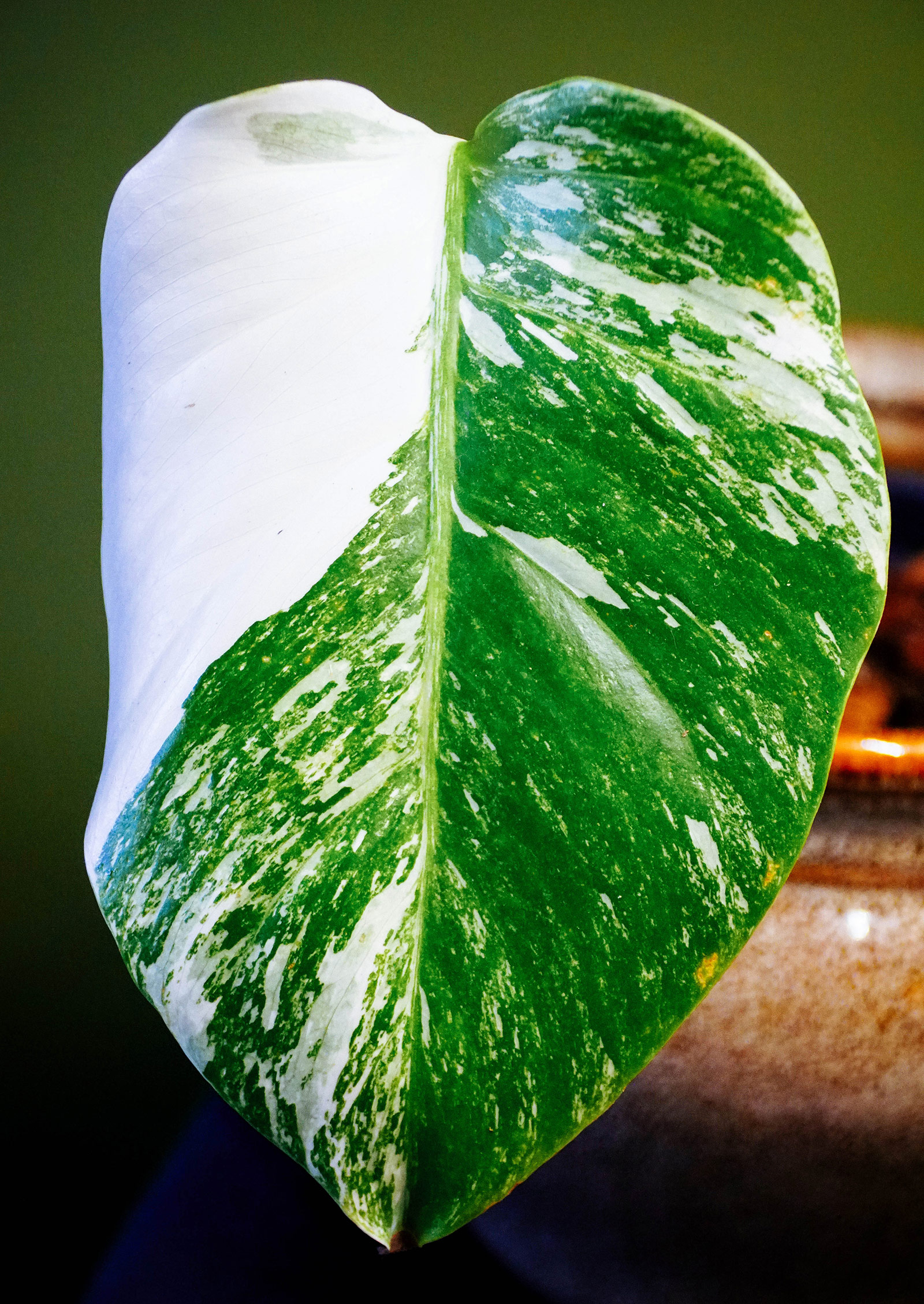The photograph captures a close-up of a large leaf with its background fully blurred, rendering a mix of green, brown, and darker shades. The leaf is divided distinctly down the middle by a very light green stem. The left half of the leaf is predominantly stark white, covering about 70% of its surface with some green interspersed beneath. This white area seems to extend from the top to roughly two-thirds down the side, and it appears almost painted. The right half of the leaf retains natural green hues, featuring various shades of green with small light green and white splotches scattered across. The leaf's texture varies, appearing thicker in some places and thinner in others. The blurred background includes hues of green and brown, possibly elements of the same leaf extended beyond the focus. The upper background corners display dark and lighter greens, while the bottom corners range from very dark, almost black tones, to patches of light blue, red, and orange, introducing a gradient of colors.